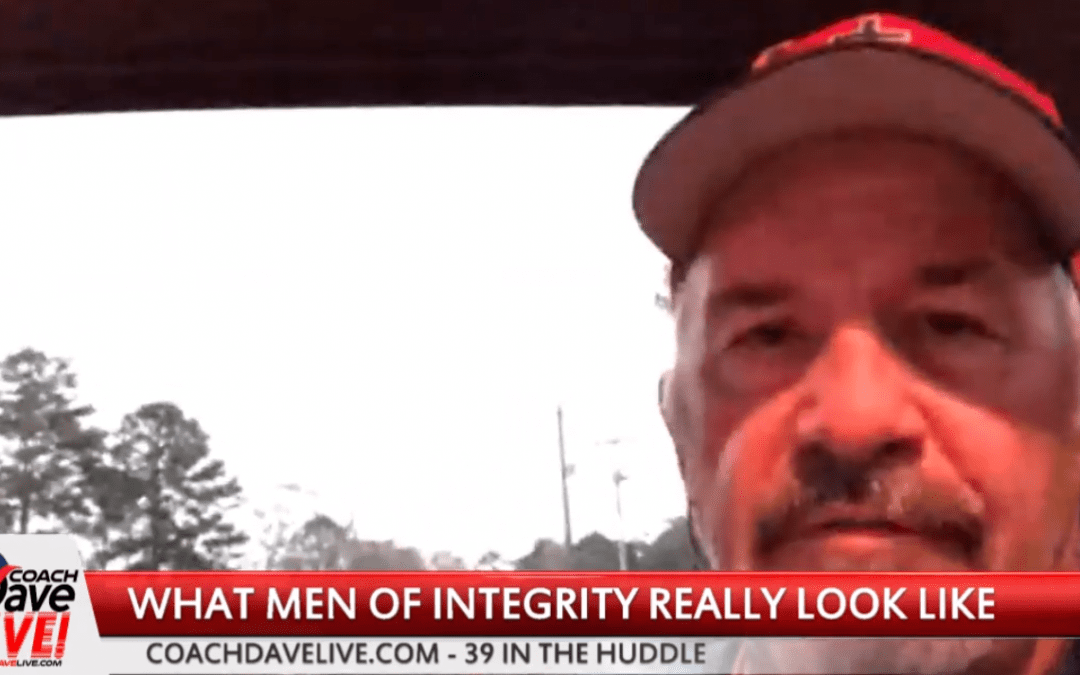The image depicts a broadcast screen from a TV network, featuring a close-up of an older, bearded man with a mustache and dark eyebrows, wearing a red cap with a white underside. He has a serious expression as he looks directly into the camera. The background is a grayish scene with visible trees, telephone poles, and possibly the top of a car. Dominating the bottom portion of the screen is a red banner with white capital letters declaring, "What Men of Integrity Really Look Like." Below this is a white banner with gray text reading "CoachDaveLive.com-39 in the Huddle." Partially cut off on the left side, a gray area reveals the text "Coach Dave Live!" with an exclamation mark, though parts of the letters are obscured.